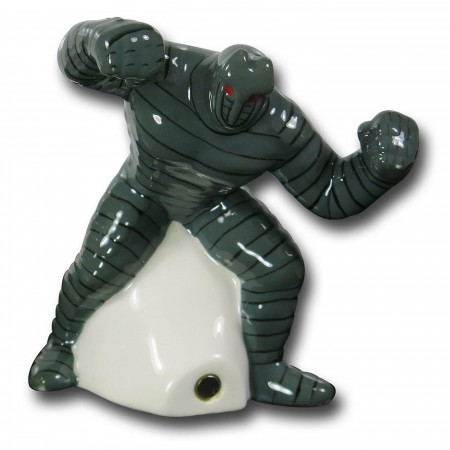The photograph captures a glossy, dark gray figurine with black stripes and striking red eyes, standing against a stark white background. The muscular humanoid figure, resembling a cross between a sumo wrestler and a mythical creature, has clenched fists raised as if poised to deliver a powerful punch, with one arm positioned for an overhead strike and the other for an uppercut. Its body, devoid of discernible facial features aside from the menacing red eyes, bends slightly forward in a combative stance. The figure's unique aesthetic includes a pattern of tightly spaced black stripes on its glossy gray surface, giving it a painted appearance. It is mounted on an off-white, stone-like base which might function as a pencil sharpener, evident from an opening at the front surrounded by metal. The entire piece casts a prominent shadow against the white backdrop, enhancing its imposing presence.